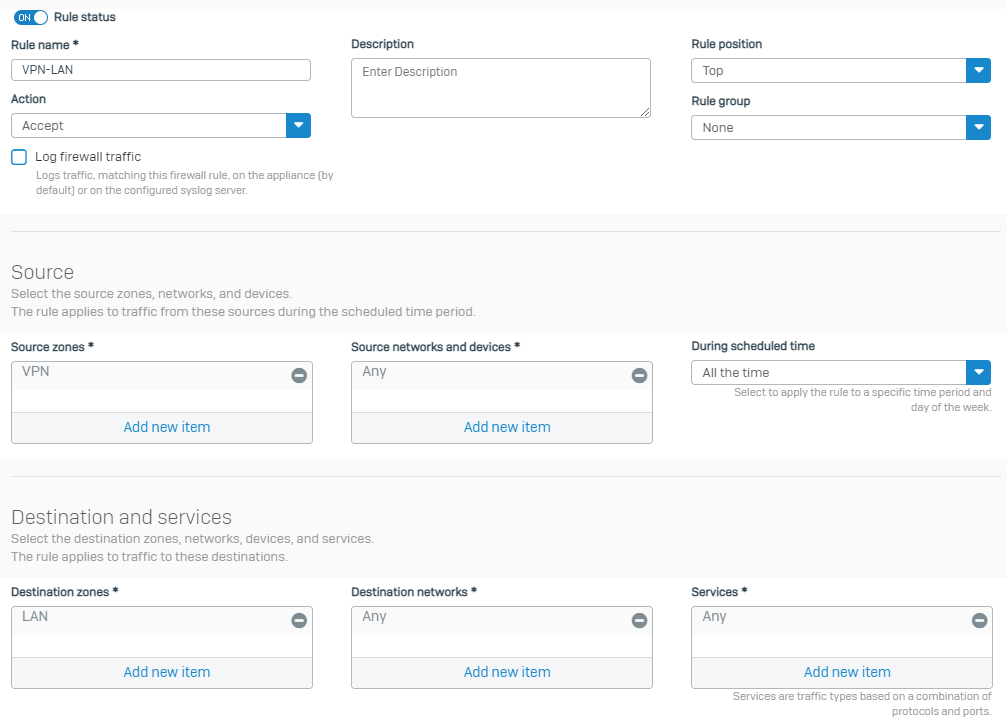This image showcases a detailed configuration page of a browser interface for setting up and managing firewall rules. At the top left corner, there is a toggle button indicating the rule's status, labeled "Rule Status." Just below, there is a field for "Rule Name" marked with an asterisk, accompanied by a text input box containing the label "VPN LAN." 

Further down, there is an "Action" line with a dropdown menu set to "Accept," and beneath this, a checkbox labeled "Log Firewall Traffic" is present. On the right-hand side, the interface includes various options, such as a "Description" box, a "Rule Position" dropdown menu pre-set to "Top," and a "Rule Group" dropdown menu showing "None" as the selected option. These dropdown boxes are stylized in blue with a downward arrow in the middle.

In the "Source" section, there are three boxes. The first box, labeled "Source Zones," displays a label "VPN" with an "Add New Item" option at the bottom, and features a minimize button at the top right corner. The second box, titled "Source Networks/Devices," contains the term "Any," also with an "Add New Item" option and a minimize icon at the top right corner. The third box, "During Schedule Time," is set to "All the time."

The "Destination and Services" section is divided into three boxes: "Destination Zones" on the left, "Destination Networks" in the middle, and "Services" on the right. This organized layout provides a comprehensive set of options for managing firewall rules effectively.